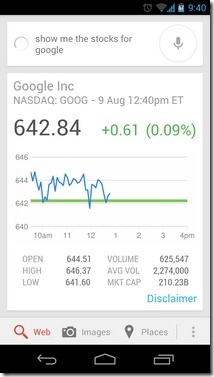This vertical rectangular image features a user interface for a stock query about Google Inc. The top and bottom sections of the image are bordered by black horizontal bars, with the bottom bar being slightly thicker. In the top right corner, a series of icons are visible.

Below the top black bar, there's a white horizontal rectangle displaying the text in gray lowercase letters: “show me the stocks for Google," next to a gray microphone icon. 

Beneath this, a larger vertical white rectangle shows the latest stock info for Google Inc. The light gray text at the top displays "Google Inc." and directly below it, the stock listing "NASDAQ: GOOG," followed by "9 AUG, 12:40 PM ET" in capitalized letters and numerical characters.

Prominently, the stock price of 642.84 is printed in bold black font. Next to it, a green font denotes a slight increase with "+0.61 (0.09%)". The accompanying graph displays a horizontal green line at 642, intersected sporadically by a jagged turquoise line representing the stock’s fluctuating performance.

Below the graph, several columns of additional stock data are listed in light gray: "OPEN: 644.51", "HIGH: 646.37", "LOW: 641.60", "VOLUME: 625,547", "AVERAGE VOLUME: 2,274,000", "MKT CAP: 210.23B". 

To the bottom right, the word "disclaimer" is highlighted in turquoise. 

Encasing the stock data, the bottom horizontal light gray bar includes more navigation options. To the left, a red magnifying glass icon with the label "web" in red or orange is seen. Following this are icons for "images" with a camera, "places" with a teardrop, all in light gray font. The bottom row houses additional icons for other functionalities.